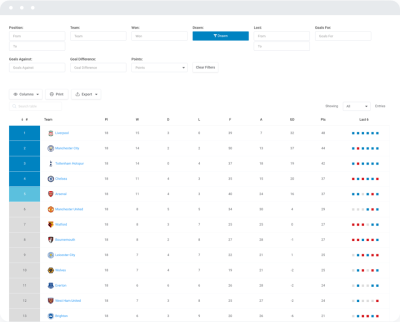This screenshot captures a ranking chart, although the text is indistinguishably small and blurry. The screenshot displays a gray bar at the top that contains the close, minimize, and expand buttons, which are not colored as typically seen on a Mac interface. Below this bar, there is a row of six fields, with one of these fields filled in blue. Following this, there are two white fields, succeeded by three more white fields and a clickable button. Further down, there are three additional clickable white buttons.

The core of the screenshot is a chart containing 12 distinct rows, possibly representing sports teams or clubs, denoted by icons and text directly to the right. There are eight columns with numbers adjacent to the names, likely indicative of rankings or scores. Towards the far right, an additional column features primarily blue dots interspersed with a few red ones, suggesting a scoring or tracking system. Despite the overall blur, this layout hints at a detailed and structured system, presumably organizing and displaying team or club-related data.